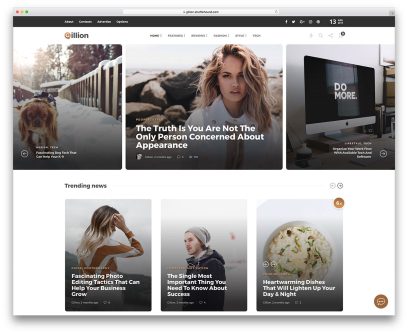This is a detailed screenshot of a user interface. At the top center, there is a white rectangle containing very small black text. Directly below this is a horizontal black rectangle with four white words on its left side and various icons on its right side. Beneath this section is a significant amount of white space, leading to a centered menu with six items. Each menu item has an icon to its right, and a company name and logo are positioned to the left.

Further down, there are three photographs. The leftmost image features a dog playing in the snow. In the middle photograph, a woman with long, dirty blonde hair stands in front of a rocky background, with a text overlay in white that reads, "The truth is you are not the only person concerned about appearance." The rightmost image displays a computer monitor with a central text in uppercase white letters that says, "DO MORE."

Below more white space, three additional photographs are centered on the page. Above these images, on the left side, bolded in black, are the words "Trending News." The first photograph depicts a woman with long blonde hair, raising her right arm to her forehead. The middle image shows a man wearing a hat and a blue coat. The rightmost photograph appears to show a white cookie.